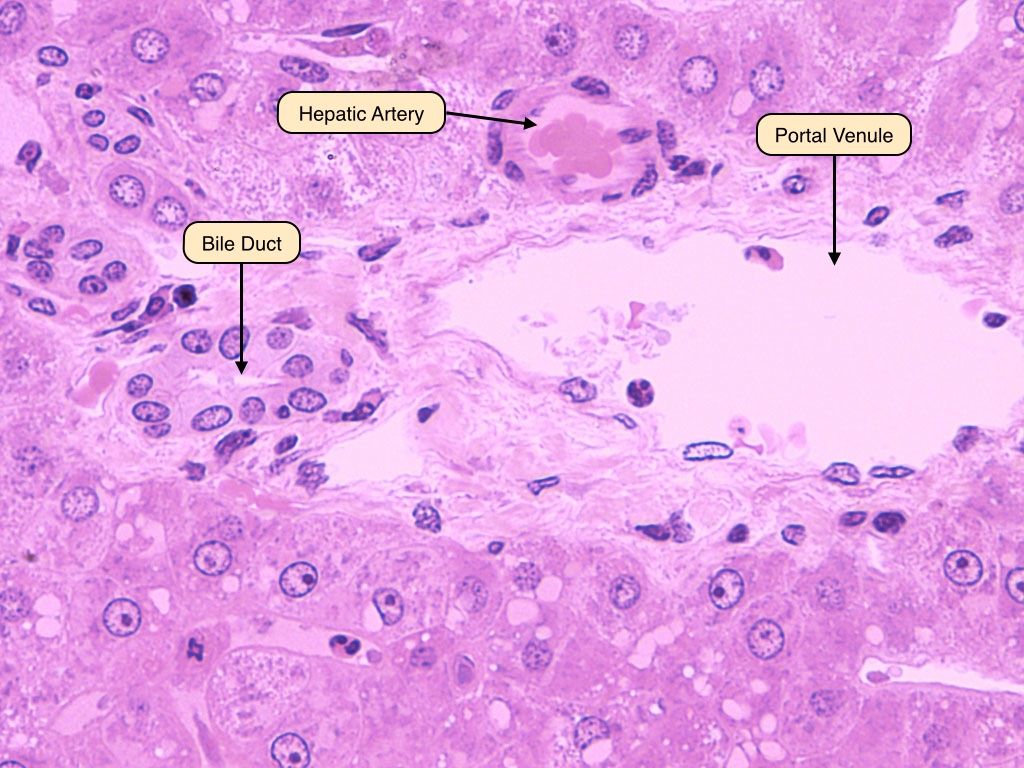This is a highly detailed microscopic image predominantly in shades of purple and pink. The image displays a series of round, dark purple ring cells, some of which contain smaller dark purple dots inside them. The arrangement suggests these could be blood cells or similar microscopic structures. There are three distinct labels in the image, each marked by an arrow pointing to specific areas. The first label reads "bile duct," the second one, positioned above and to the right, says "hepatic artery," and the third label, situated to the right of the "hepatic artery," states "portal venule." The labels are written in black text within yellow bubbles, providing a clear identification of these anatomical features.